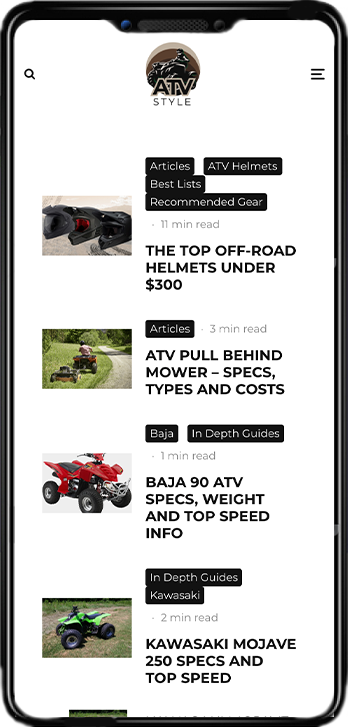The image depicts a mobile screen displaying a webpage dedicated to ATV articles and guides. The edges of the mobile phone are visible and black, while the screen itself is white. On the top left corner is a search icon resembling a magnifying glass, and on the top right are three stacked lines representing the menu.

At the center of the screen, there's a heading that reads "ATV Style," accompanied by a logo featuring a person riding an ATV. Below this, a list of article previews is presented. The visible articles include:

1. **Top Off-Road Helmets under $300:** A detailed list article, 11-minute read, featuring an image of three black helmets placed on a gray cement surface.
   
2. **ATV Pull-Behind Mower Specs, Types, and Costs:** A brief, three-minute read article with a photo of a person riding an ATV, pulling a mower behind, mowing grass beside a road.
   
3. **Baja 90 ATV Specs, Weight, and Top Speed Info:** A one-minute read guide, described as an in-depth guide.
   
4. **Kawasaki Mojave 250 Specs and Top Speed:** A two-minute read article, another in-depth guide.

The last article's title is partially cut off, indicating there are more articles to browse through below the screen's visible area.